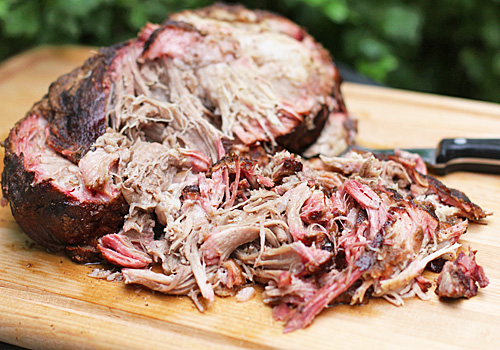This close-up photograph showcases a partly cut beef roast, resting on a wooden cutting board, adorned with intricate engravings along its edges. The succulent roast, likely pulled from a smoker given its crusted and seared exterior, exhibits a beautiful spectrum of colors: the outer crust comprises shades of dark brown and light brown, while the interior ranges from deep reds and pinks to light browns and beige. The board, situated outdoors as hinted by the dark green foliage and the natural daylight, enhances the rustic charm of the scene. To the right of the meat, partially obscured by the roast, lies a black-handled carving knife, marked with a silver rivet. The overall composition, complete with sunlight cascading down, suggests an intimate outdoor culinary session.